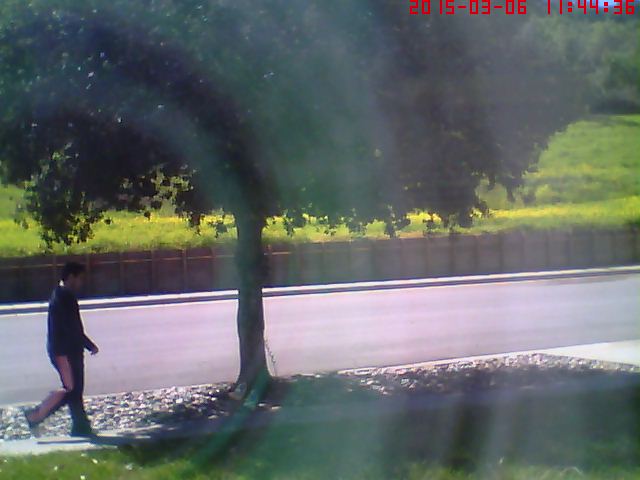This photograph, possibly a still from security footage, has a slight distortion potentially caused by being taken through glass. It captures a scene looking out onto a road, with a tree prominently in the foreground, accompanied by a sidewalk and a patch of grass – likely part of someone's front yard. Beyond the road, a fence stands before a vast grassy area extends into the distance. A person with light skin and dark clothing is walking along the sidewalk, facing to the right. In the upper right-hand corner of the image, a timestamp in red letters reads "2015-03-08 11:44:36," indicating the date and time the photo was captured.